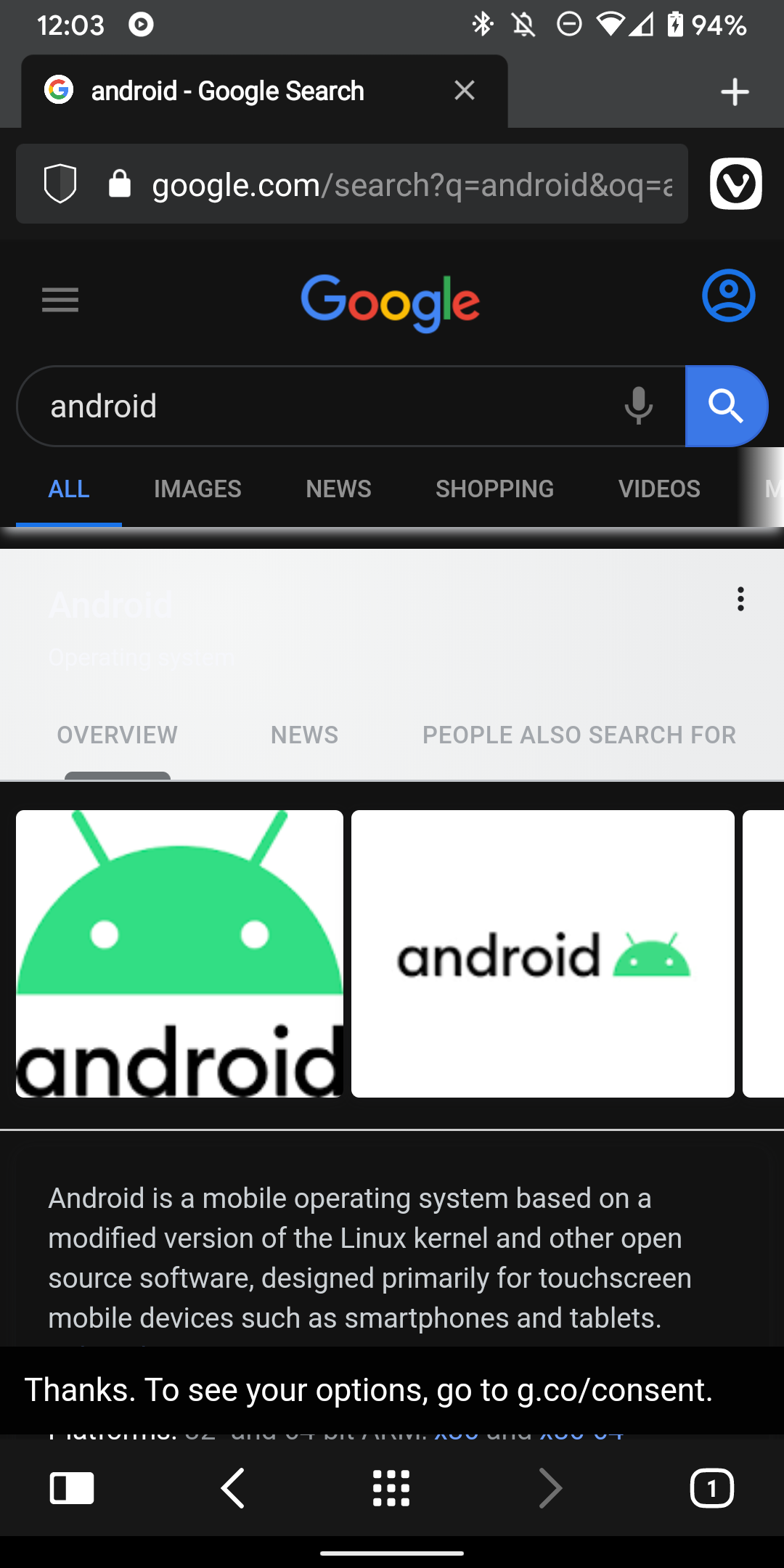A detailed caption for the image:

"The screenshot displays a Google search page on an Android device at 12:03 PM with a battery level of 94%. The search query appears to be 'Android', as indicated by the underlined 'All' tab in blue within the search categories, which include Images, News, Shopping, and Videos. The interface shows typical Google search navigation features like the magnifying glass icon for search and the microphone icon for voice search. 

Below the search bar, the page highlights tabs such as 'Overview,' 'News,' and 'People also search for.' The 'Overview' section provides detailed information stating that 'Android is a mobile operating system based on a modified version of the Linux kernel and other open-source software, designed primarily for touchscreen mobile devices such as smartphones and tablets.' Additionally, there is a prompt suggesting options for user consent on Google's policies with a link, 'go to g.co/consent'.

At the bottom of the page, there are several navigation icons: a white rectangle with a smaller black rectangle inside it, an arrow pointing left, an arrow pointing right, a grid of nine circles, and a number '1' enclosed in a square."